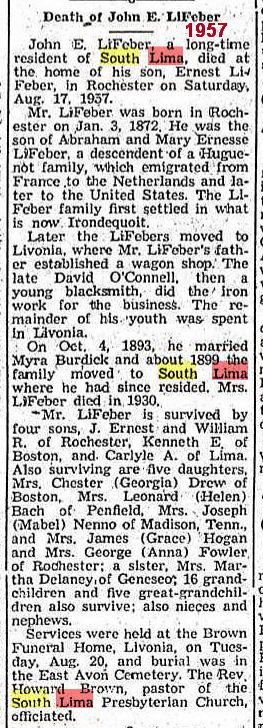This image depicts an obituary printed in a newspaper, formatted in column style with black text and certain words highlighted in yellow and red. It commemorates the life of Johnny Lee Feber, a long-time resident of South Lima, who passed away on Saturday, August 17, 1957, at the home of his son, Ernest Lee Feber, in Rochester. Born on January 3, 1872, in Rochester, Johnny was the son of Abraham and Mary Ernest Lee Feber, descendants of a Huguenot family that emigrated from France to the Netherlands before settling in the United States. The Lee Feber family initially established themselves in what is now Irondequoit, later moving to Livonia where Johnny's father opened a wagon shop, with the ironwork done by a young blacksmith, David O'Connell. Johnny spent his formative years in Livonia, marrying Myra Burdick on October 4, 1893, before relocating to South Lima around 1899, where he remained until his passing. Myra Burdick Lee Feber predeceased him in 1930. Johnny is survived by his children, including sons J. Ernest and William R. of Rochester, Kenneth E. of Boston, and Carlisle A. of Lima; and daughters Mrs. Chester (Georgia) Drew of Boston, Mrs. Leonard (Helen) Bach of Penfield, Mrs. Joseph (Mabel) Ninmo of Madison, Tennessee, and Mrs. James (Grace) Hogan and Mrs. George (Anna) Fowler of Rochester. He is also survived by his sister, Mrs. Martha Delaney of Geneseo, 16 grandchildren, 5 great-grandchildren, along with numerous nieces and nephews. Funeral services were conducted on Tuesday, August 20, at the Brown Funeral Home in Livonia, with burial following at the East Avon Cemetery. The service was officiated by Reverend Howard Brown, pastor of the South Lima Presbyterian Church.